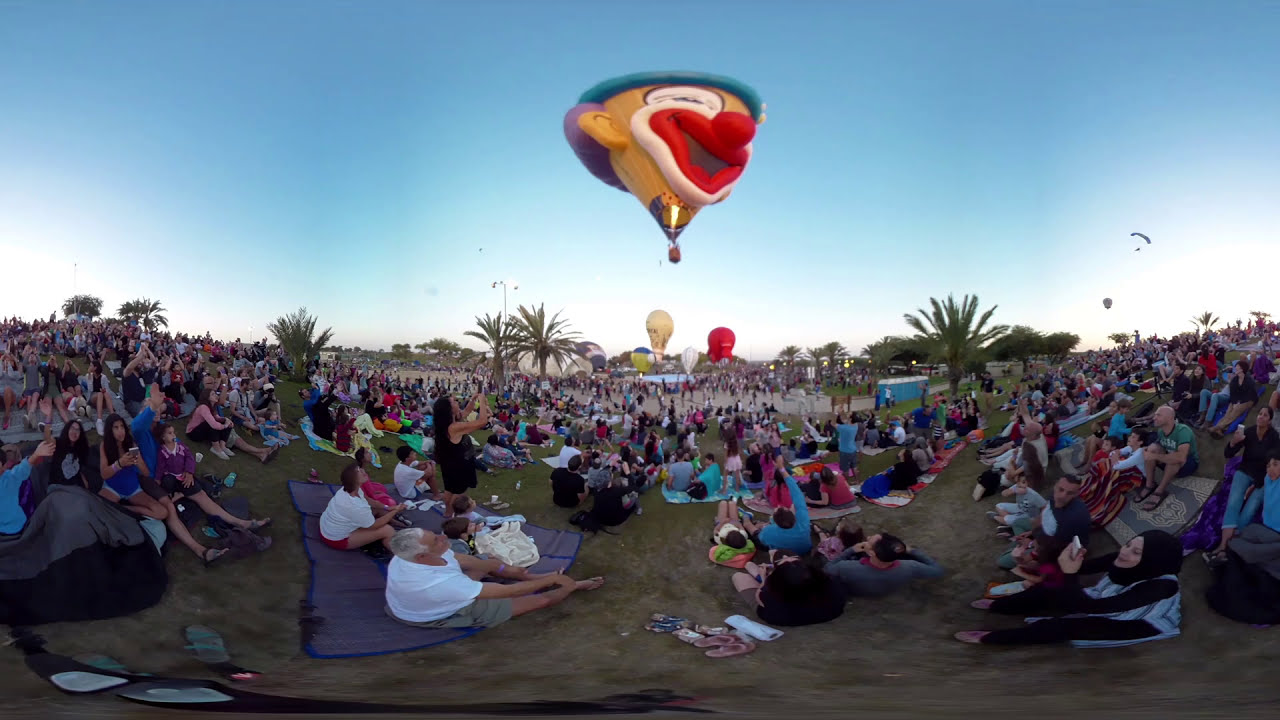The image captures a vibrant balloon festival on a clear, bright day with blue skies. The grassy field forms the base of the photograph, dotted with palm trees and crowded with hundreds, if not thousands, of people of various ages, backgrounds, and cultures. These spectators are either seated on colorful blankets, in chairs, or directly on the grass, collectively facing the sky to watch the spectacle. In the center of the panoramic shot, a whimsical hot air balloon resembling a clown's head ascends, drawing attention with its yellow skin, purple hair, red mouth, and white-lined red lips, all topped with a green cap. Flames are visible in the basket below, providing the lift. Surrounding this clown balloon, several other hot air balloons are also preparing for take-off. Off to the side, the scene extends to a plaza area with shops, lights, and porta-potties, underscoring the event's festival nature. The overall atmosphere is lively and colorful, with hues of blue, white, purple, yellow, teal, and red dominating the scene.